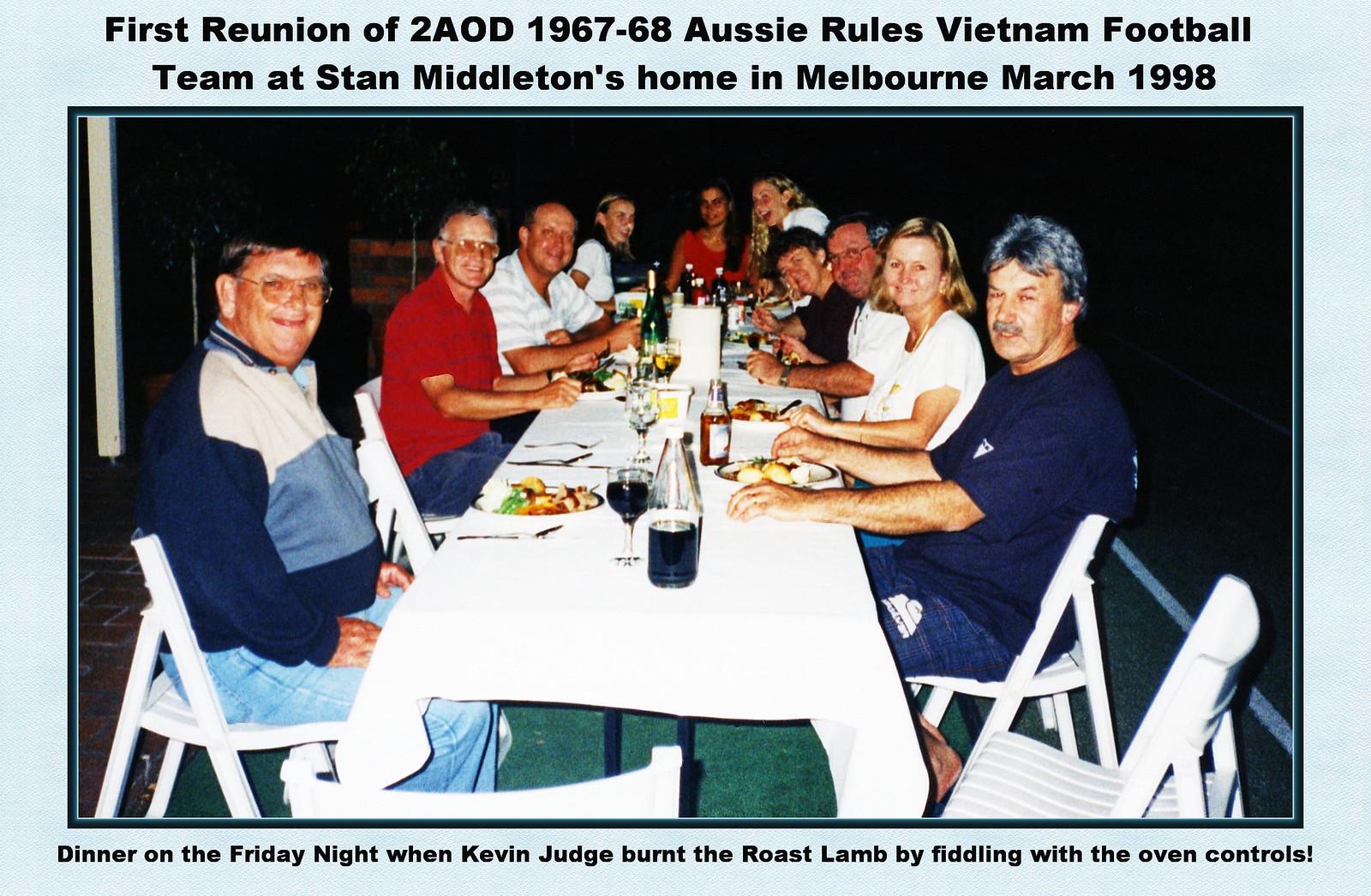The image captures the first reunion of the 2AOD 1967-68 Aussie Rules Vietnam football team at Stan Middleton's home in Melbourne in March of 1998. The reunion dinner took place on a Friday night, notably remembered for when Kevin Judge burnt the roast lamb by fiddling with the oven controls. The photograph, bordered in blue, frames a long, white tablecloth-covered table set outside on what appears to be a deck or balcony under the night sky. A large group of predominantly middle-aged, Caucasian individuals is gathered around the table, all smiling and engaged. They are casually dressed in relaxed clothing, comprising mainly of blue jeans, and many are wearing tinted glasses. The table is laid with plates, utensils, bottles of wine, sodas, and beers, signifying an enjoyable feast. On the left side of the table, four adults are seated, mirrored by five adults on the right, and a woman at the head of the table. The woman at the head is in a red top with long brown hair, flanked by individuals in various casual outfits. The scene conveys a jovial and laid-back atmosphere, filled with camaraderie and shared memories, against a backdrop that confirms it's nighttime.